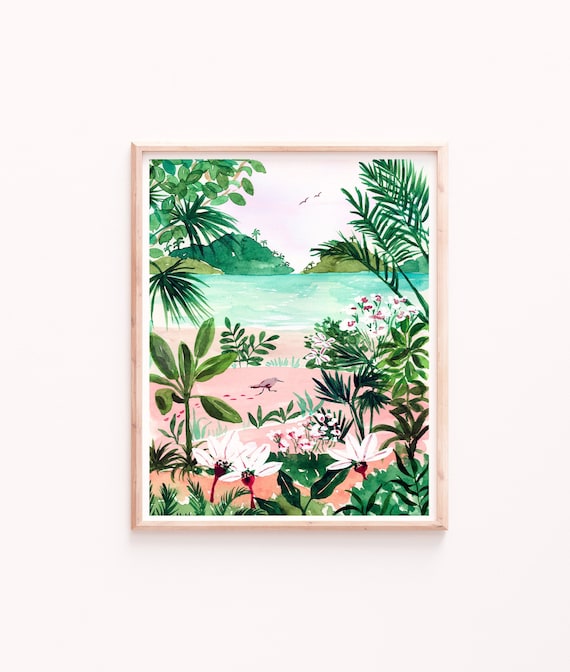This detailed product image is designed for commercial use, ideal for an online shop, listing, or catalog. The overall shape of the image is rectangular, with the left and right sides being twice the length of the top and bottom sides. The background emulates a light pink wall, providing a staged and somewhat artificial appearance. Mounted on this wall is a piece of artwork framed in a light brown natural wood frame, also rectangular with the same side proportions.

The frame encompasses an inner white border, drawing attention to the vivid drawing it surrounds. The artwork itself is an exquisite depiction of a tropical island scene. The foreground features pink beach sand where a small pink bird can be seen, its footprints trailing behind. Scattered around are various tropical plants with lush green leaves, including some that resemble ferns and a few smaller flowering plants. These flowers have red centers and pinkish-white petals.

The middle ground of the scene reveals a serene body of turquoise blue water, painted with a natural stroke. Beyond the water, to the right, rise several islands shaded in green, dotted with palm trees, evoking a lush and vibrant landscape. The sky above is open and clear, with two birds in flight adding a sense of freedom and movement to the scene.

Overall, this painting captures a tranquil tropical environment, framed in a light brown wooden frame and set against a pinkish background, perfect for showcasing in a commercial setting.